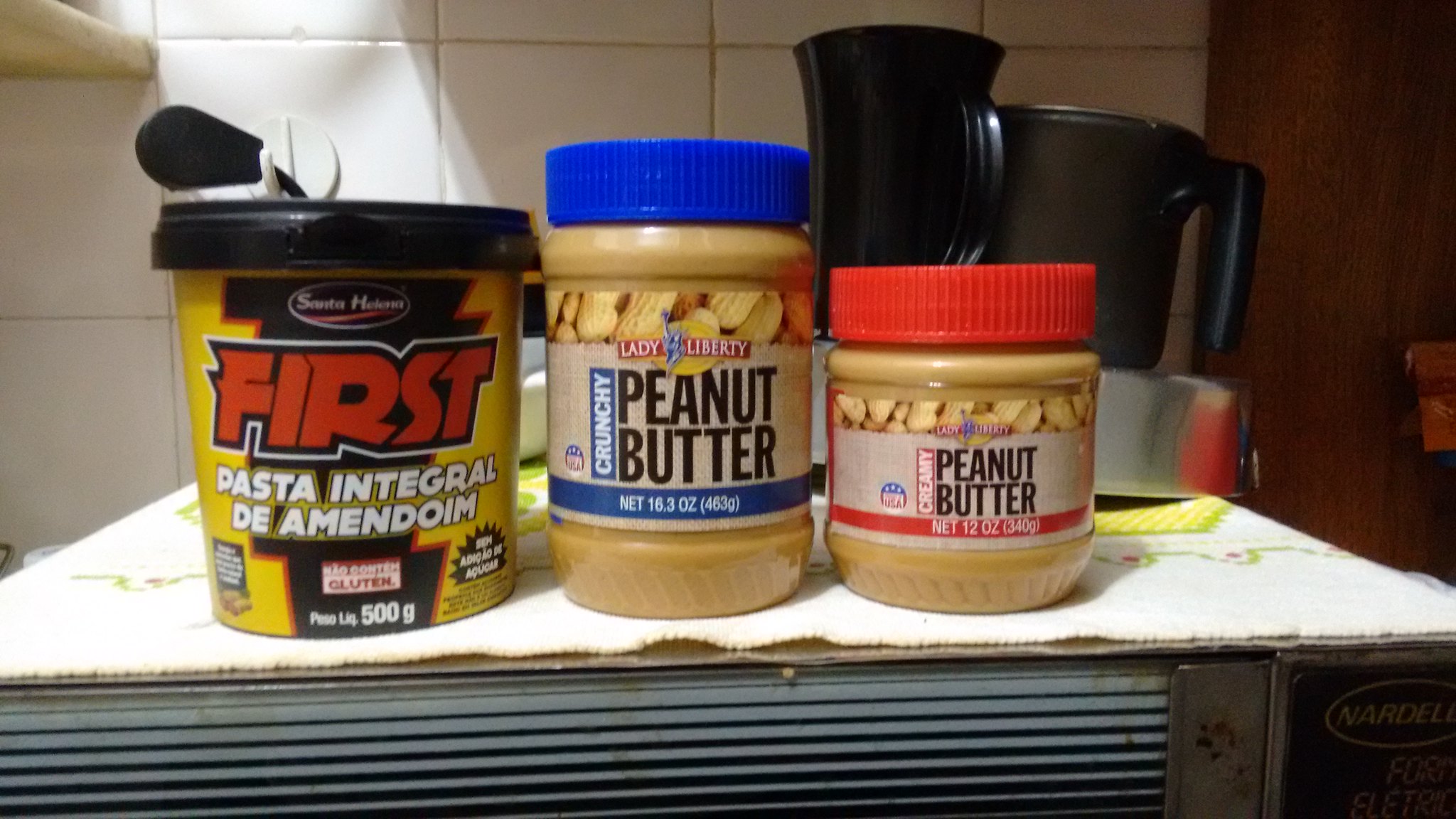In this clear, color photograph, three jars, predominantly of peanut butter, are meticulously arranged in what appears to be a kitchen or a hotel room. The jars rest on a white towel, which is likely placed on a heater or an AC unit, evident from the visible white grid of the appliance beneath and some grey and white horizontal lines. In the background, a coffee maker and possibly a kettle or some mugs are noticeable against a grey tiled surface and a window ledge with sunlight streaming in from the upper left.

The central jar is a larger, blue-capped, crunchy peanut butter with a beige label featuring a blue stripe at the bottom indicating its weight. To its right, a smaller jar with a red cap contains creamy peanut butter. Its label displays an image of peanuts and annotations such as "Lady Liberty" at the top and “peanut butter” in black, with details of its weight, "12 ounces 340 grams," written in red at the bottom.

On the left, the jar has a black cap and stands out as possibly not peanut butter but another spread, labeled "Santa Helena." The text on this jar reads "First Pasta Integral D Amendium" with a black, red, and white color scheme. The collection of jars is garnished by the warm lighting and domestic ambiance of the room, making them the focal point against a backdrop that includes subtle kitchen elements and a soft play of sunlight.